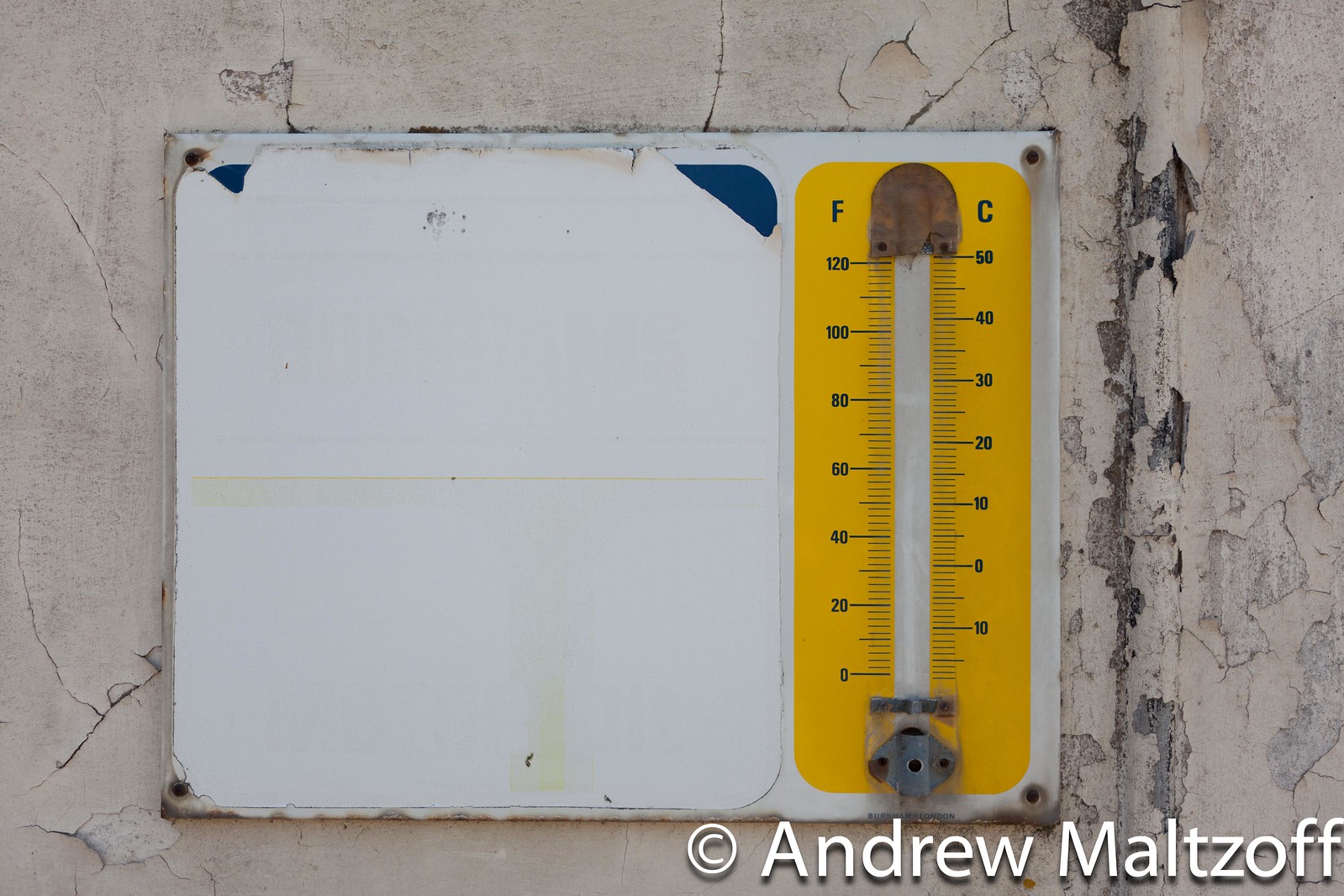This photograph features a weathered and chipped gray plaster wall. The wall, showing significant wear and tear, exhibits numerous chips and marks. Towards the right side of the image, a notable crack is visible, transitioning to a darker black shade due to accumulated dirt and grime. Mounted on the wall is a white rectangular plaque, which appears to be secured at the corners by screws. A hint of blue is visible in one of the corners of this plaque. Adjacent to the plaque is a vertical yellow measuring device, likely a thermometer. At the top of the thermometer, the letters "F" and "C" are printed in black, indicating measurement in Fahrenheit and Celsius, respectively, with numbers running down the length of the device.

In the bottom right corner of the image, there is a copyright symbol "©" followed by the name "Andrew Maltzoff" written in white text.